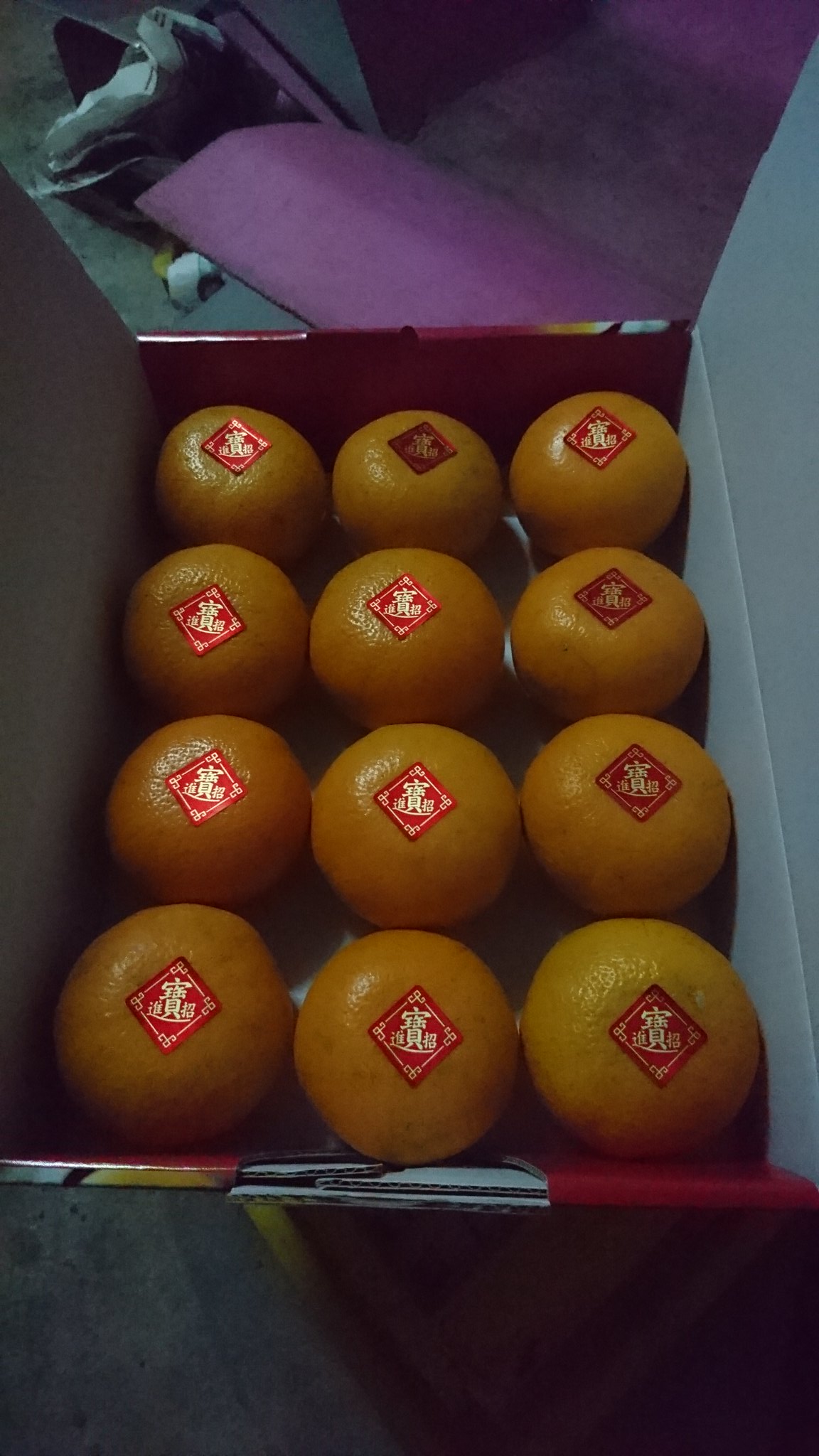The indoor color photograph captures a neatly arranged box of twelve ripe and bright orange tangerines. The tangerines are organized in three precise columns of four, making for an orderly and appealing presentation. Each fruit bears a square label in the center, decorated with red and Japanese white lettering, suggesting they are from a Japanese company. The box itself is white with hints of red and yellow decorations on the visible side, and it has two flaps on top that can be folded over for sealing, transforming it into a practical shipping container. In the background, there is a hint of pink packing material. The overall scene is slightly dark, with the foreground particularly dim. The tangerines appear fresh, well-placed, and free from any signs of damage or insect infestation, making them look ready for display or shipment.